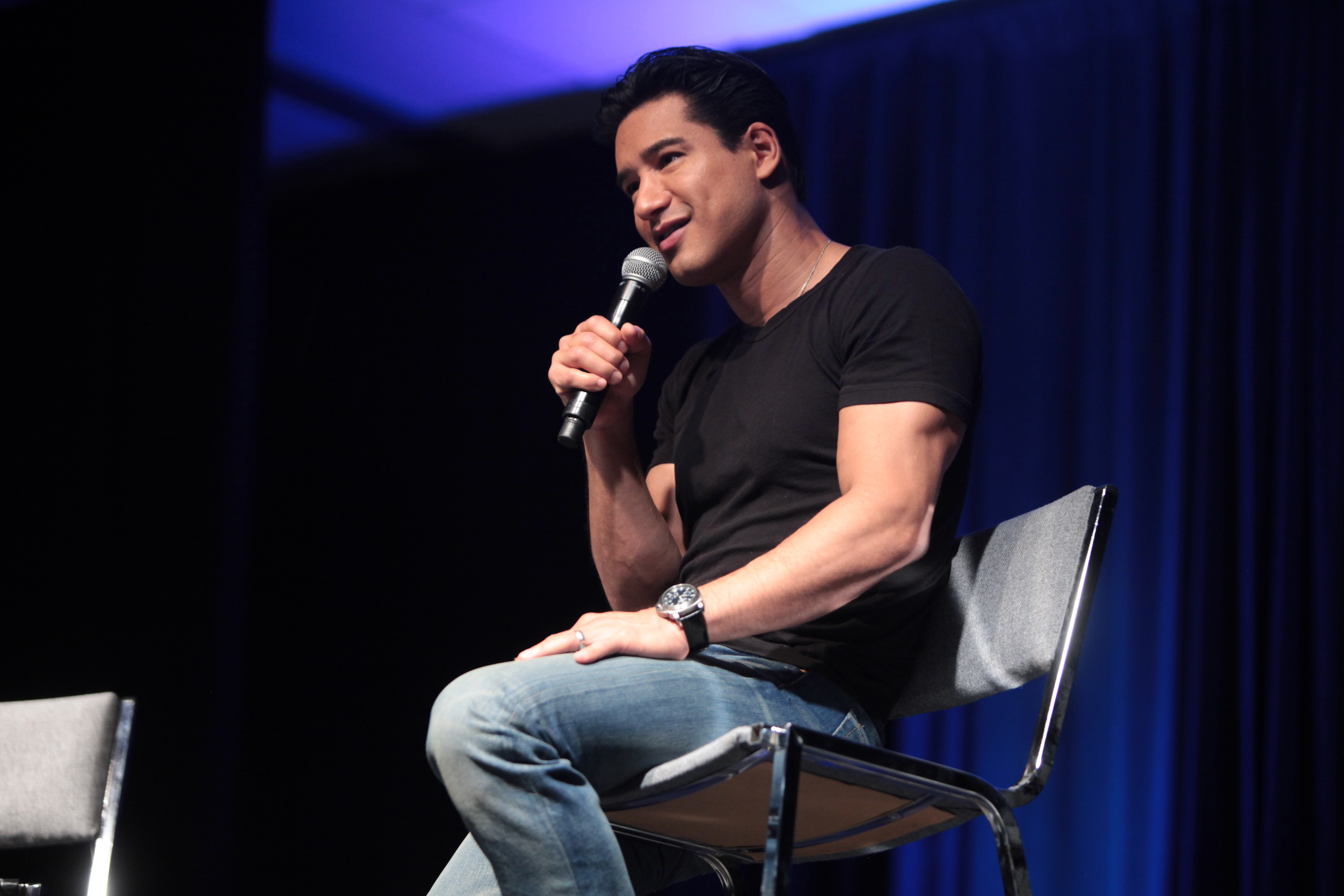This photograph features actor Mario Lopez seated on a metal-framed chair with a gray back and cushion, akin to those found in waiting rooms or offices. He is casually dressed in a black short-sleeve t-shirt and light blue jeans. On his left wrist, he sports a sleek watch with a silver face and black strap. Lopez is holding a black microphone in his right hand and appears to be speaking, directed toward the left side of the image as though he is engaged in conversation or addressing an audience. His short, slicked-back dark hair complements his muscular build. The backdrop consists of large blue curtains, and to his left, the top half of an identical chair can be seen. Above him, the ceiling features a triangular design that transitions from dark to lighter blue hues.